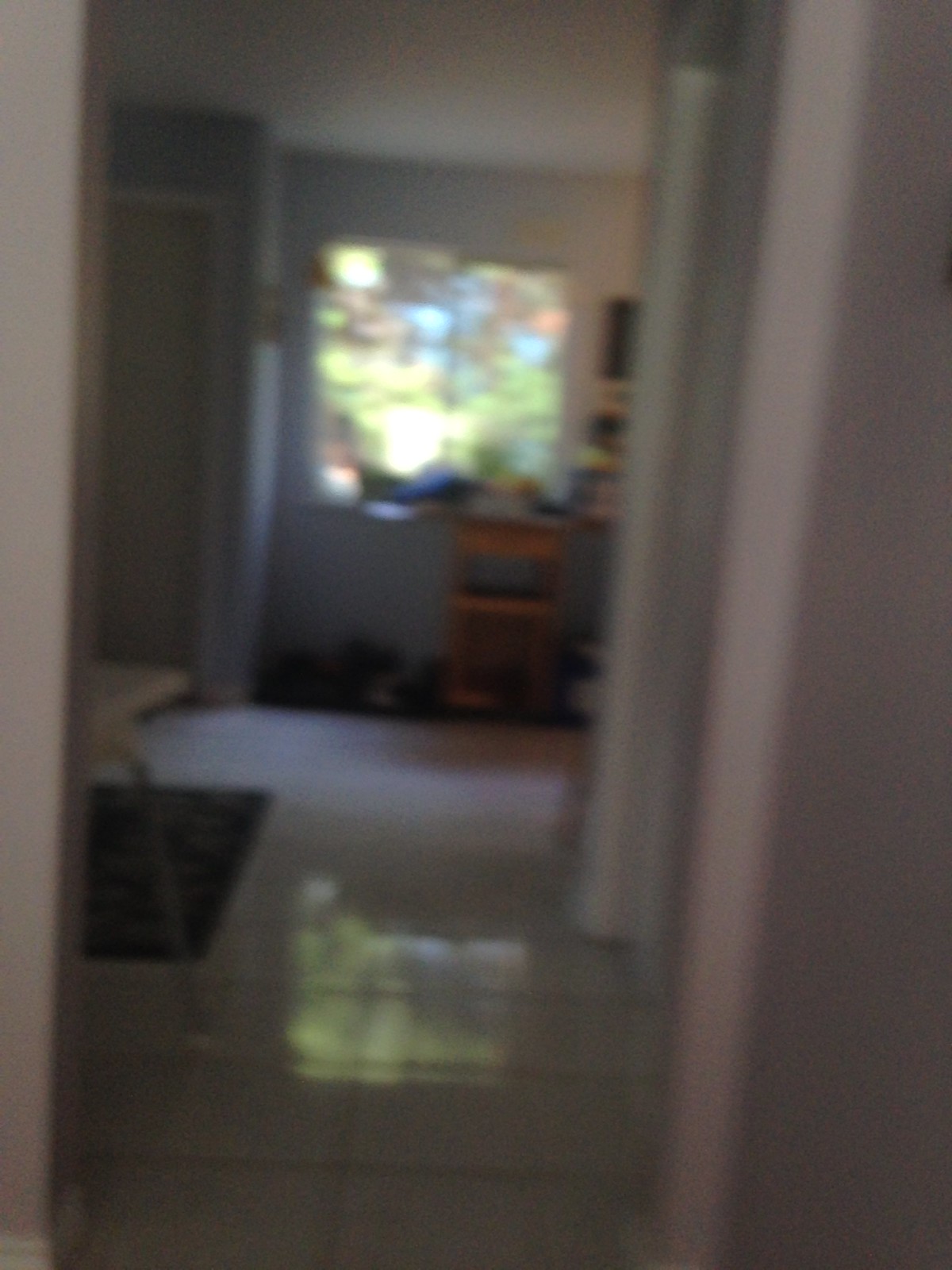The blurred image depicts a small living space, likely a cozy home or an apartment. The main room visible in the photo houses what appears to be a brown chair, possibly sized for a child, suggesting the room might be a child's play area. The window in view offers a glimpse into what could be the child's room. The background, though blurry, suggests an outdoor environment under sunny conditions, featuring some indistinct greenery, possibly bushes, in a backyard setting.

Within the room, there are noticeable items scattered on the shiny, white floor tiles, which could be shoes or pieces of clothing, predominately black in color. The left side of the image reveals a door, while the right side hints at another door frame and what might be a wall. Additionally, there's a black rug, and a corner of a cream-colored cocktail table with a visible leg, contributing to the cozy, lived-in feel of this home.